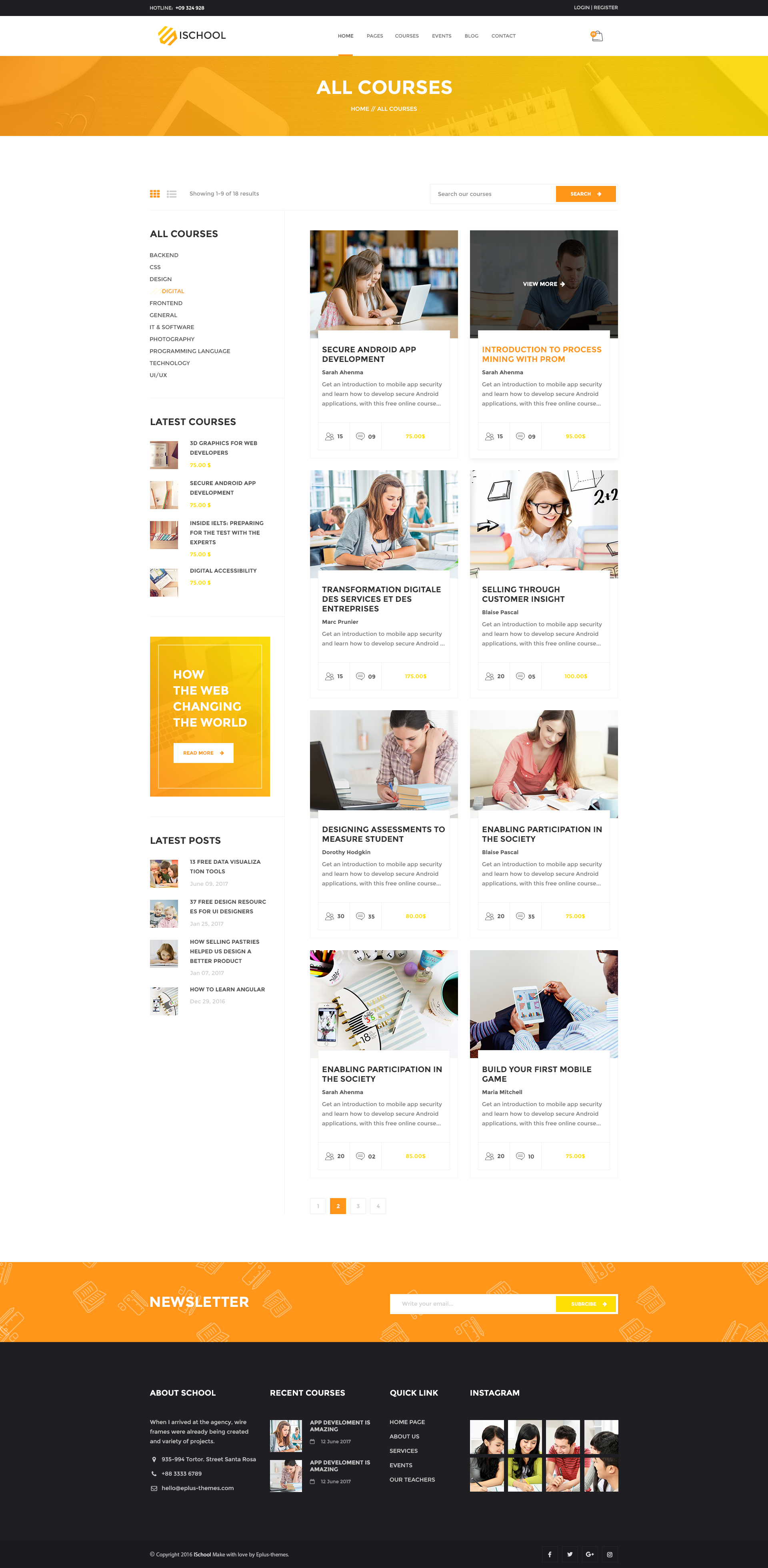The screenshot depicts a desktop view of a detailed website's homepage, specifically for an educational platform named "iSchool." The web address, browser, and operating system details are not shown. 

At the very top of the page, there is a black bar displaying a hotline number "09324928" on the left in white text, and "Login or Register" options on the right, also in white text. Below this, prominently positioned, is a yellow hexagon logo featuring the word "iSchool," with the "i" styled as an igloo.

The navigation menu beneath the logo includes options for Home, Pages, Courses, Events, Blog, and Contact, alongside an icon of a shopping bag displaying a numeric indicator. The Home page is currently highlighted. 

A yellow banner stretches across below, featuring icons reminiscent of a notebook, a pen, and a snippet of a phone screen. This section offers the ability to toggle the view between grid or list formats for search results, which are currently displaying 1 to 9 out of 18 total courses.

On the left sidebar, there are categories like "All Courses," "CSS Design," "Digital" (highlighted in orange), "Front End," "General," "IT and Software," "Photography," "Programming Language," "Technology," and "UI/UX." 

The main section showcases various courses with associated images, mostly depicting people in educational settings. Course titles include "Secure Android App Development," "Introduction to Process Mining with PROM," "Transformación Digital en Empresas," "Selling Through Customer Insight," "Designing Assessments to Measure Student Learning," "Enabling Participation in Society," and so forth. Each course card provides details such as the instructor's name, class size, or comment count.

To the right, there's a section for the latest courses and posts, featuring articles like "How the Web Changed the World." At the bottom of the page, users can sign up for a newsletter, view quick links (Home, About Us, Services, Events, Teachers), and see the most recent courses, one of which dates back to June 12, 2017.

The footer includes the contact information for the iSchool headquarters located at 935 to 994 Tortor Street, Santa Rosa, with a phone number of 883-333-36789 and an email address "hello@plus-themes.com." A copyright notice for the year 2016 states "iSchool made with love by E Plus Themes," accompanied by social media icons for Facebook, Twitter, Google Plus/Google Hangouts, and Reddit.

This image captures either a work-in-progress or an already active educational website designed for course browsing and enrollment.